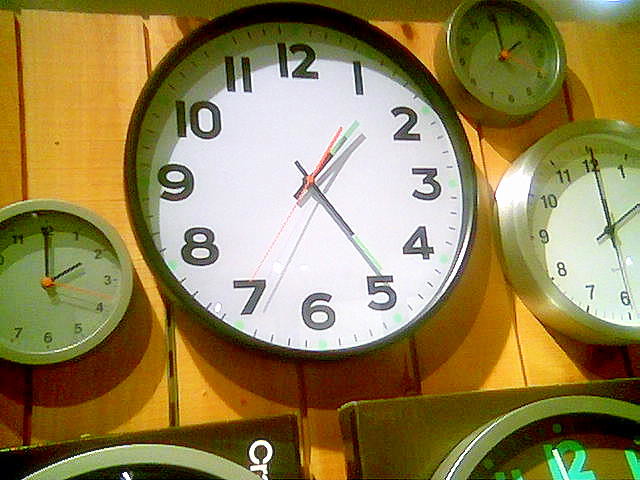This photograph features a wall adorned with a variety of clocks mounted on a panel with a wood texture. The centerpiece is a large, round clock with a white face. To its right, there is a medium-sized clock with a white face and a smaller clock, both of which are green. To the left of the central clock, there is another small green clock. Below these central timepieces are the tops of two additional large clocks set within wooden square frames. The clock on the bottom right is distinguished by its green numbers and white hands. The clock in the bottom center section sports a white face, a red second hand, and black minute and hour hands that have white tips. The overall composition of the wall creates a visually engaging mosaic of different clock designs and sizes, all unified by the wooden background.